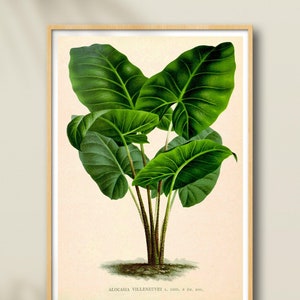Hanging on a silky-looking wall, this framed illustration captures a plant with striking detail. The light brown, thin wooden frame encloses a central image of an elephant ear plant, set against a beige or creamy peach background. The plant features six to seven large, dark green leaves that transition to a lighter green towards the edges. These leaves emanate from a central stem that starts brown at the base and gradually lightens as it ascends. Below the plant, there's some illegible text, likely indicating the plant's name or species. The ground around the base of the plant is illustrated in a dark brown.